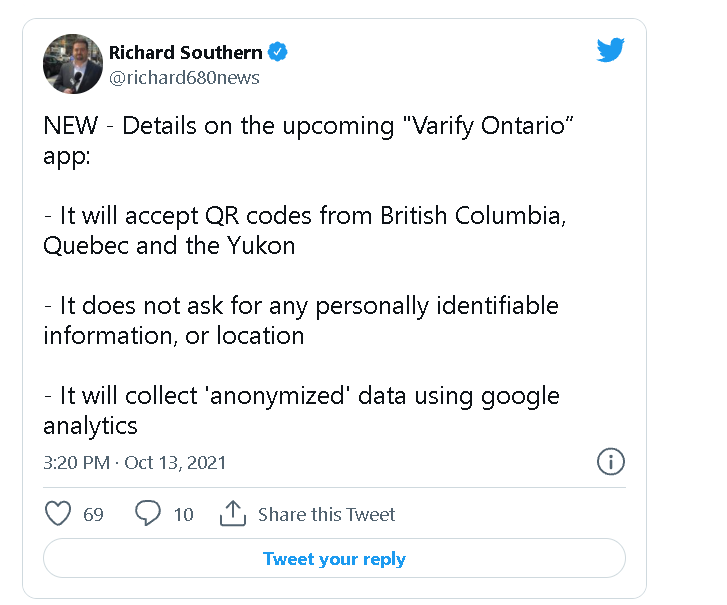Here is the cleaned-up and detailed caption for the image:

---

The image is a screenshot of a tweet by Richard Southern, a verified Twitter user indicated by a blue checkmark. His Twitter handle is @richard680news. The upper right corner of the tweet features the iconic blue bird symbol for Twitter.

The tweet, posted at 3:20 PM on October 13th, 2021, provides new details about the upcoming "Verify Ontario" app. According to Richard Southern, the app will accept QR codes from British Columbia, Quebec, and the Yukon. Additionally, the app will not request any personally identifiable information or location data. Instead, it will collect anonymized data using Google Analytics.

The tweet has garnered 69 likes and 10 replies. Below the tweet, options to share or reply to the tweet are available.